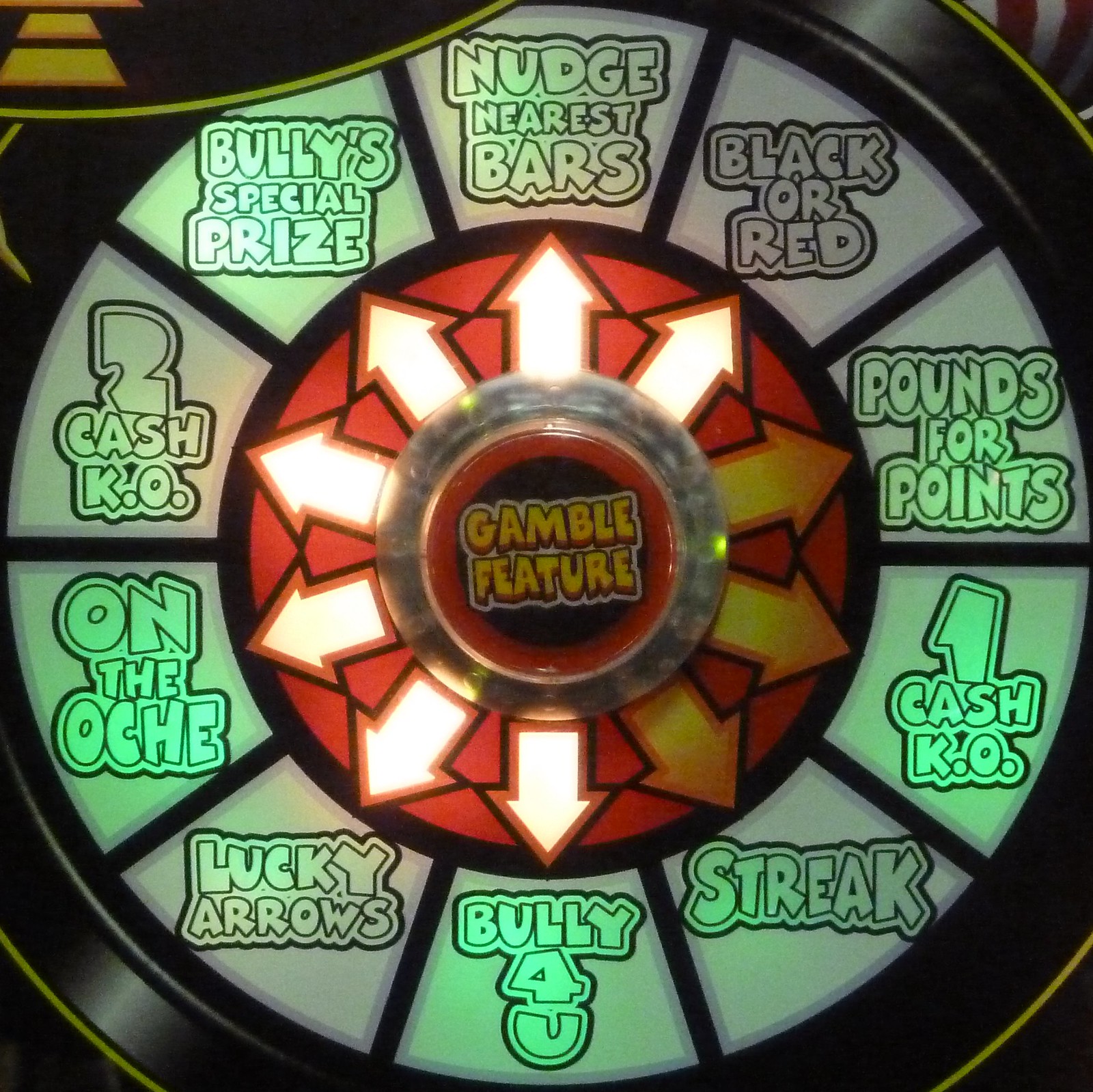A detailed photo depicts a digital game device that's reminiscent of a clock, designed for gambling or game show use. The circular design features an orange center labeled "Gamble Feature," with this area illuminated. Surrounding the center are ten illuminated arrows that point toward various segments on the outermost ring of the device. Each segment features a brightly lit, square-ish section with text indicating different game outcomes, including "Nudge Nearest Bars," "Black or Red," "Pounds for Points," "1 Cash K.O.," "Streak," "Bully for You," "Lucky Arrows," "On the Oche," "2 Cash K.O.," and "Bully Special Prize." The arrows and sections light up, suggesting that pressing the "Gamble Feature" button makes the arrows select an outcome randomly, similar to spinning a wheel on a game show.